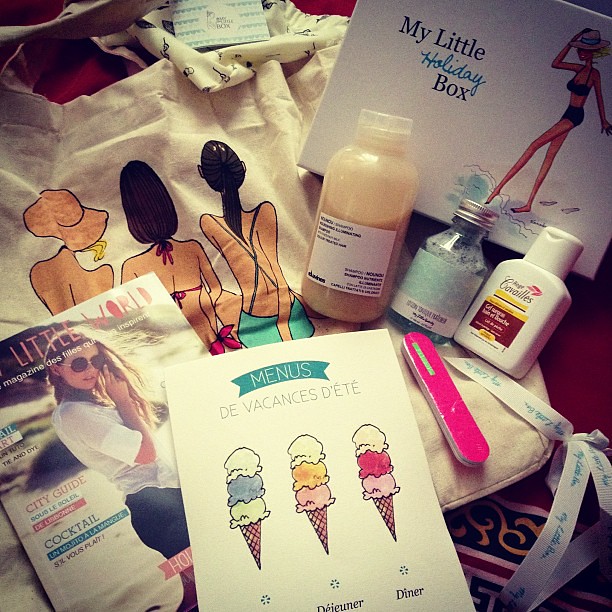This image depicts an assortment of feminine health and fashion items, carefully arranged with a yellow indoor lighting hue. Dominating the top right is a white box labeled "My Little Holiday Box," adorned with a cartoon illustration of a woman in a bikini and straw hat strolling on a beach. Below this, three blurry bottles potentially containing lotions or sunscreen are aligned next to a red or pink nail file. 

Central to the arrangement is a white card featuring a drawing of three ice cream cones, each with three colorful scoops, and labeled with menus and French text. Adjacent to this is a magazine named "Little World," showcasing a woman in a white blouse and black skirt, standing on a beach. The magazine also includes phrases like "City Guide" and "Cocktail." 

At the bottom of the image sits a cloth bag, decorated with a cartoonish depiction of three women in swimsuits, seen from behind as they sit on the beach. The overall composition of items suggests a curated gift collection themed around holiday relaxation and beauty.